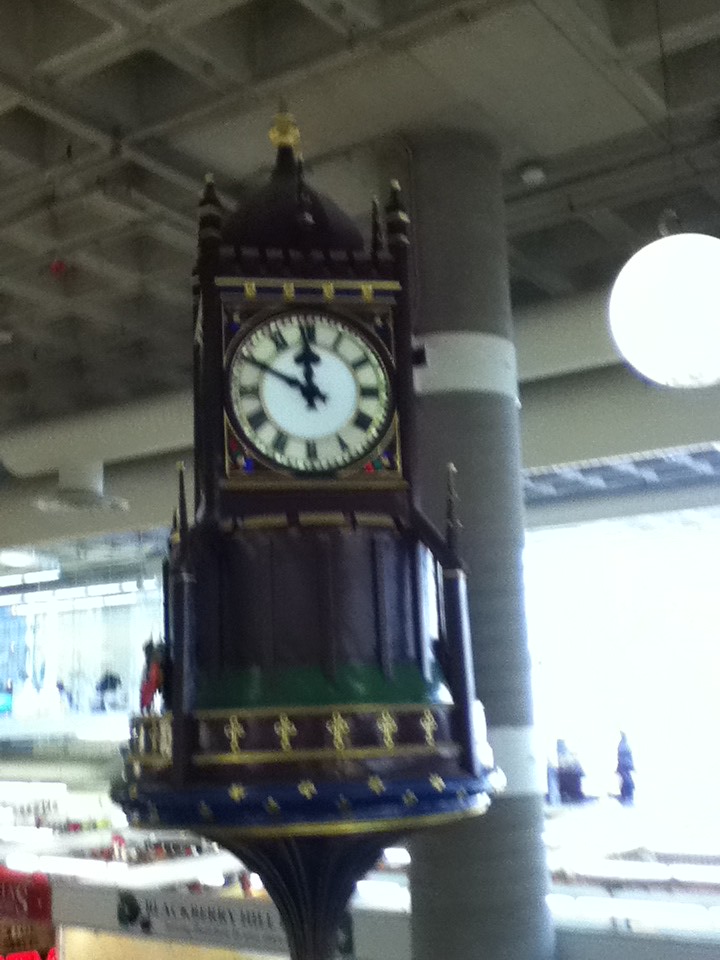The photo captures an ornate clock set within a public space that has the characteristics of both indoor and outdoor elements, such as a mall or a train station. The clock is embedded in a highly decorative mini tower structure made of dark mahogany wood, featuring intricate details that evoke a cathedral-like feel. It displays the time as 11:50 with black hands and Roman numerals on a white clock face. 

The tower hosting the clock is adorned with a series of intricate embellishments including gold crosses along the bottom and a spiral of spindles reaching up toward a black dome atop, capped with a golden ornament. The base of the structure includes several layers with different colors: brown, green, gold with red accents, and finally gold with blue fleur-de-lis patterns, growing wider as they descend. The entire arrangement narrows towards a deceptively thin base that supports it.

The background is brightly lit, suggesting daylight streaming in from what could be large windows or an open-air environment. A concrete ceiling with a dark gray, gridded pattern, and a large metal pillar supporting it, dominate the upper section of the photo, indicating the area might be an open market or public concourse with an overhead structure. There's also a conspicuous black wire, likely providing power to a circular bulb light hanging towards the right side of the image. Additionally, there is a sign mounted below the clock, hinting at a possible two-story setup. The presence of people in the background emphasizes the clock's setting in a busy, public space.